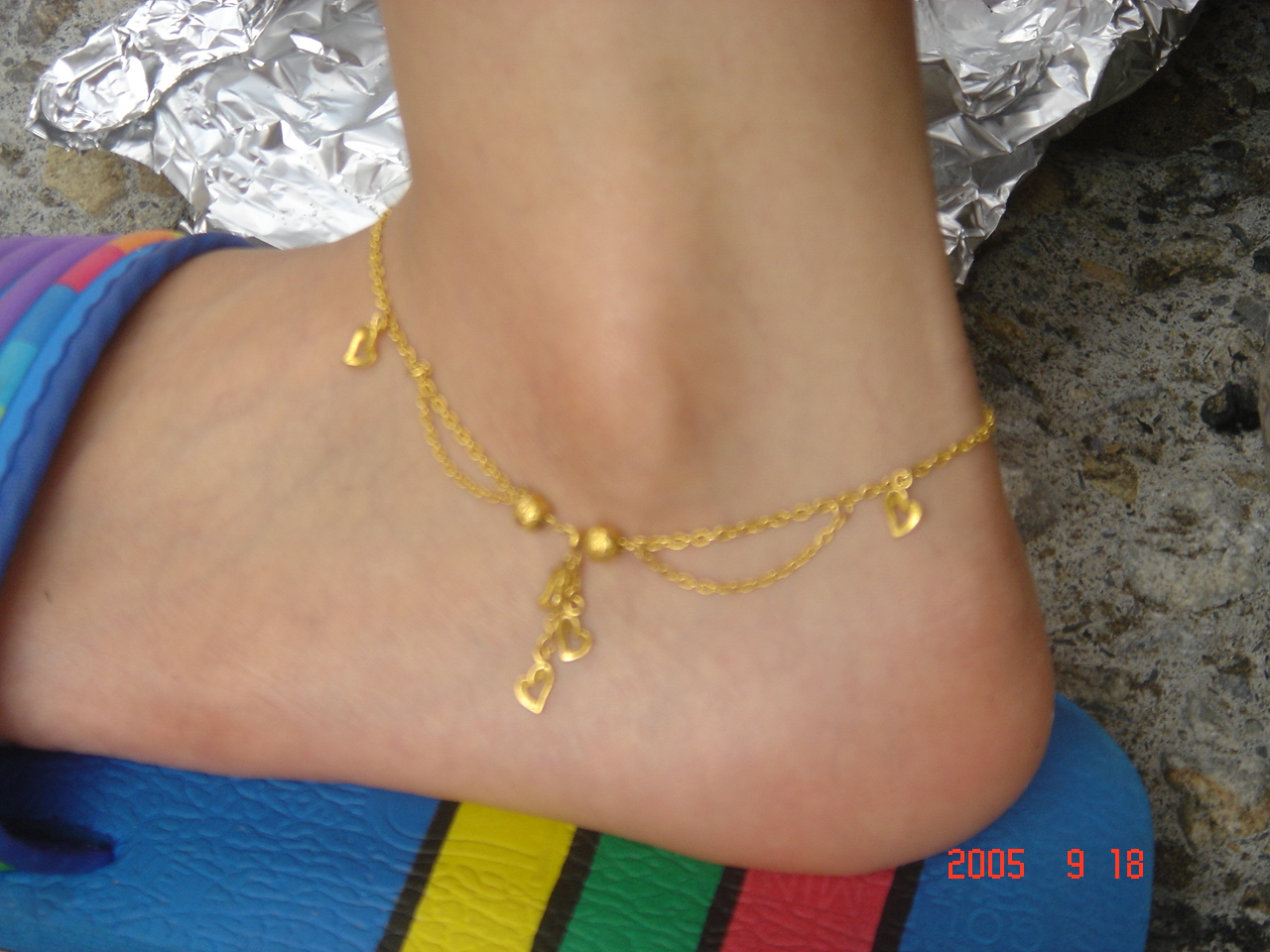This photograph, taken on September 18, 2005, clearly captures a close-up of a woman's foot adorned with an intricate golden ankle bracelet. The bracelet features delicate hanging hearts and small ball ornaments, adding a touch of elegance. The foot is clad in a distinctive blue sandal, characterized by vibrant yellow, green, and red stripes, each divided by fine black lines. The photograph notably excludes the toes, instead focusing on the ankle and heel, showing a light skin tone with visible veins. In the background, the foot rests on a possibly concrete surface, marred with discolored marks, alongside a curious piece of aluminum foil. The date "2005-9-18" is imprinted in the bottom right corner, reaffirming the photo's capture date.